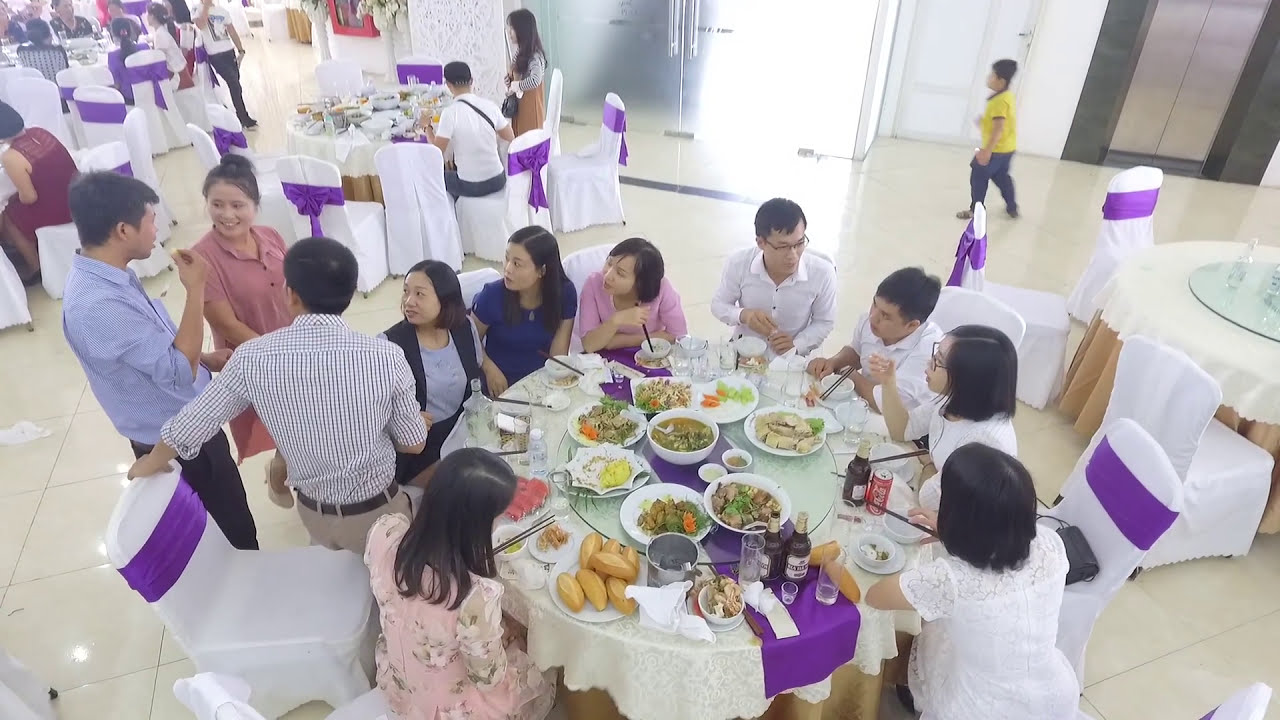The image captures a vibrant gathering in a banquet hall, likely for a special celebration such as a wedding or ceremony. The room is adorned in a white and purple theme, with circular tables draped in white tablecloths and topped with purple table runners. The chairs are covered in white cloth with purple sashes tied around the back. The atmosphere is lively with people, predominantly of Asian descent, either sitting at the tables piled with family-style dishes or standing and engaging in animated conversations. One notable person on the left, wearing a blue striped shirt, is speaking with his hand close to his mouth, drawing the rapt attention of individuals at his table. Amidst the crowd, a child, possibly around 10 or 12 years old, is seen walking alone, dressed in a yellow shirt and black pants. The background features additional tables and a stainless steel appliance, potentially a refrigerator, along with an elevator, indicating the spaciousness and multifaceted use of the banquet hall. Overall, attendees are enjoying their meals with chopsticks, savoring various dishes and drinks, creating an overall joyful and festive ambiance.